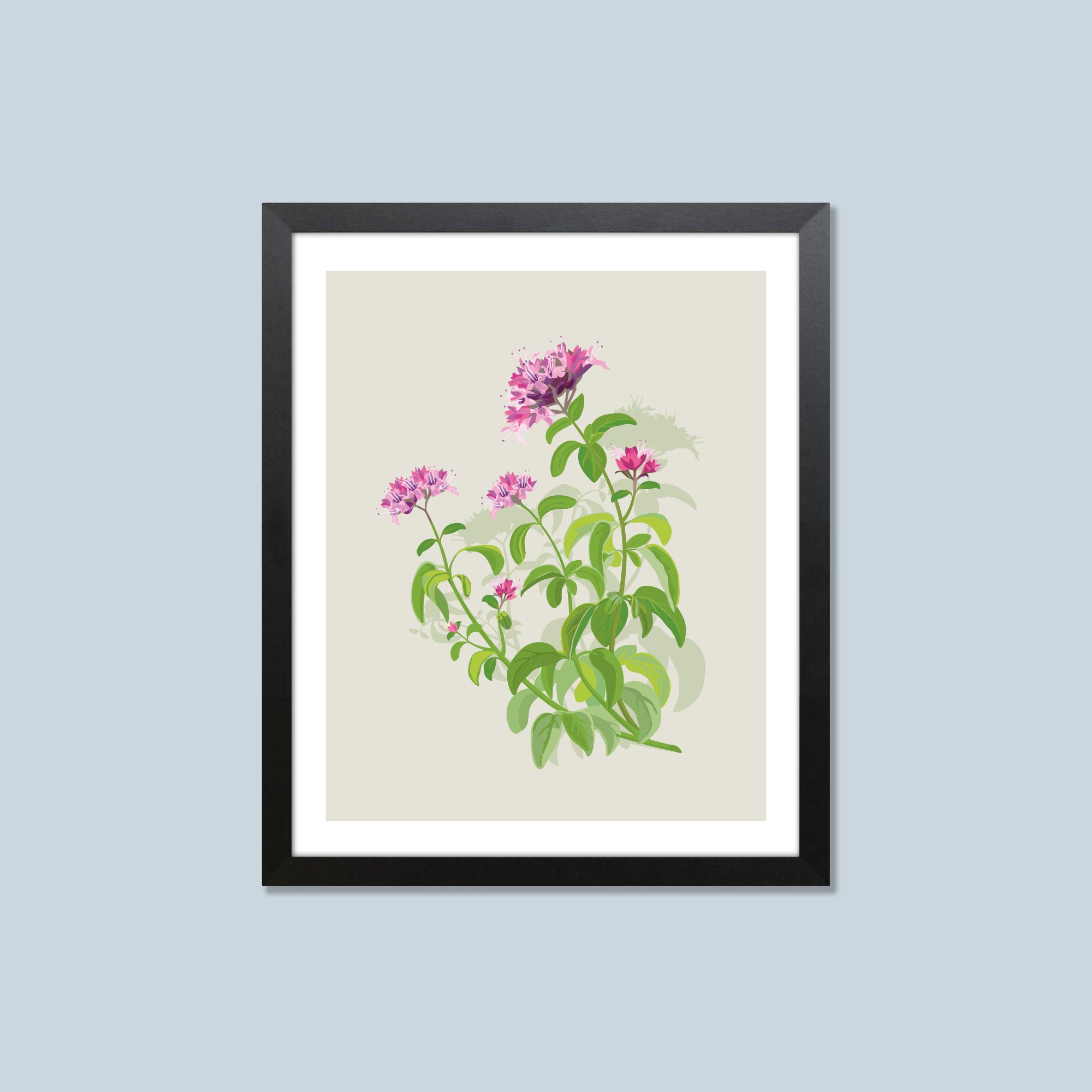This photo showcases a captivating piece of wall art prominently displayed on a light grayish-blue wall. The artwork is elegantly framed with a contrasting black frame, accented with a white mat that creates a striking double border effect. The central image features a botanical portrait on a creamy beige background. The plant depicted has a single stem with lush green leaves extending from it, each intricately detailed. The stem culminates in a cluster of six densely packed flowers, adorned with petals in shades ranging from soft pink to vibrant purple, with hints of white and red. The flowers vary in size, with the largest positioned at the top. Subtle shadows cast by the plant add depth to the image, enhancing the realism of the leaves and petals. In this serene and detailed composition, the delicate interplay of light and shadow lends a sense of dimensionality, making the floral elements stand out elegantly against their refined backdrop.